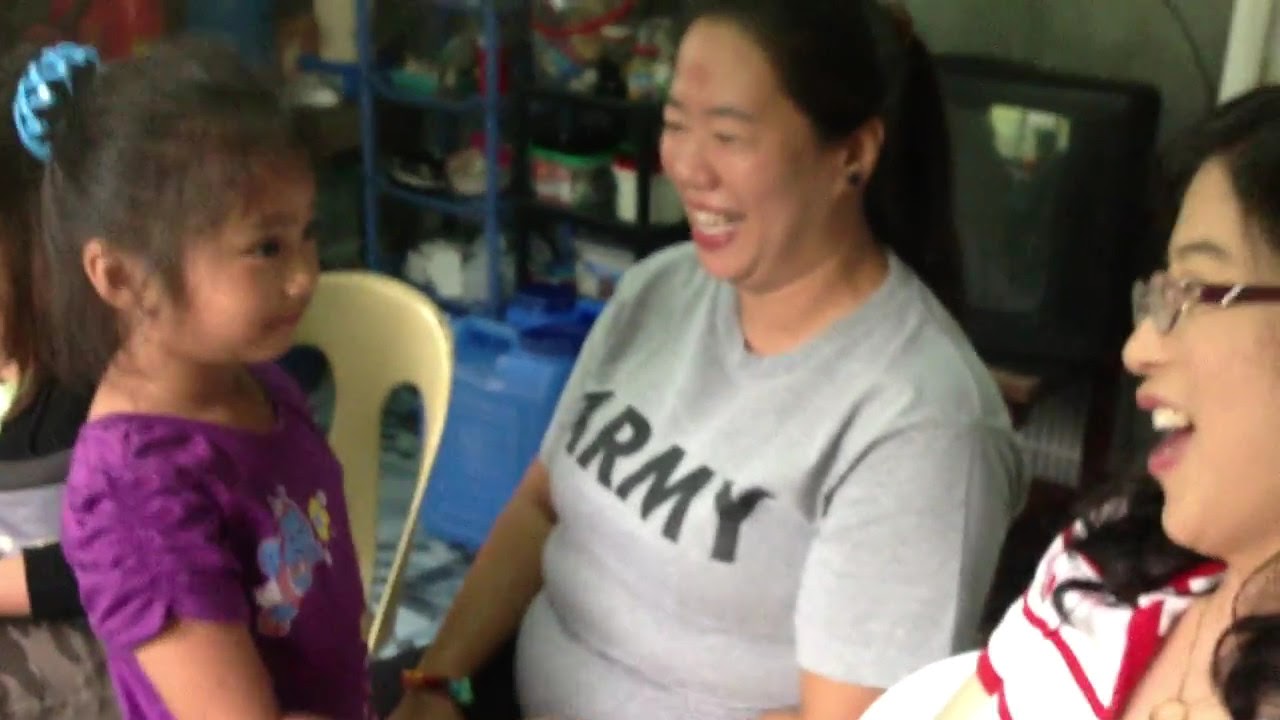In this indoor image, which appears to be taken in a preschool or a home setting, we focus on three people. To the left, there is a young Asian girl, around seven or eight years old, with her hair pulled back into a ponytail held by a light blue scrunchie. She wears a royal purple T-shirt adorned with what seem to be small character illustrations, possibly resembling a blue elephant though it's a bit indistinct. The girl faces right and appears somewhat nervous.

To her immediate right, a woman—possibly her mother or a close relative—is centered in the photo, smiling warmly. She wears a gray shirt with the word "ARMY" prominently displayed in bold black capital letters. Her hair, nearly black, is also pulled back into a ponytail, and she has black earrings.

On the far right stands another woman in glasses, dressed in a white shirt with red stripes. She, too, is smiling and looking at the young girl, while her head and posture are angled towards the left.

The background features a cream-colored plastic chair and some shelves laden with various products, as well as a TV positioned in the top right corner. This snapshot is likely taken indoors during the daytime, in what could be a living room. The scene captures a touching, familial moment, with the two women and the girl sharing a connected gaze.